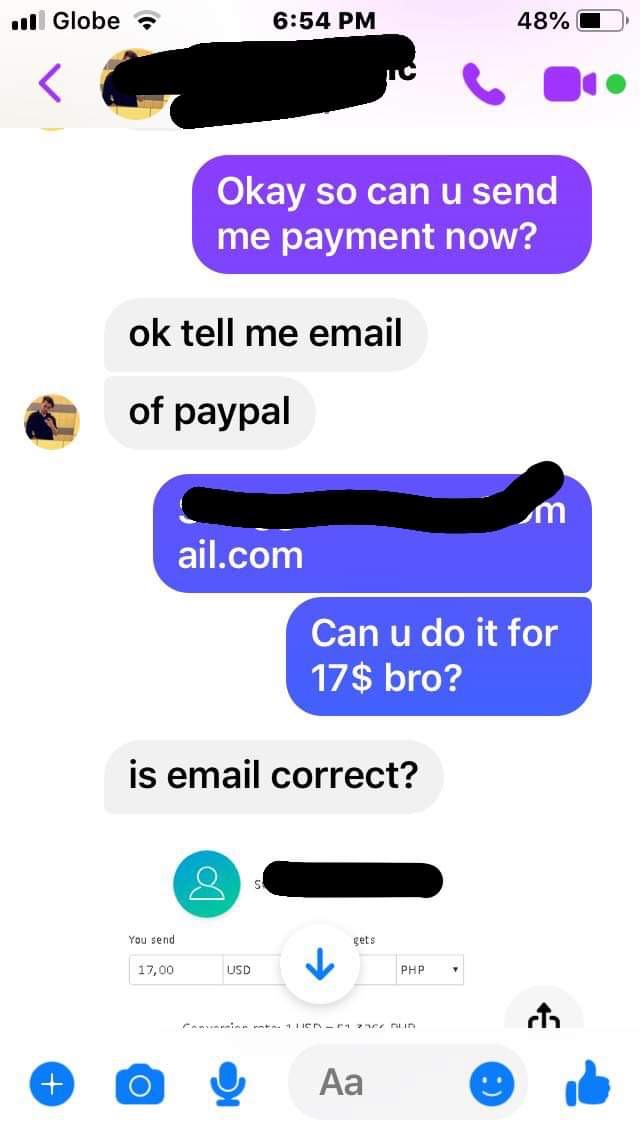This image is a detailed screenshot of a text conversation on a smartphone featuring a white background. The screen displays various indicators, including the battery level at 48%, the Wi-Fi signal, and network reception bars, with the time showing 6:54 p.m. The messages are color-coded to distinguish between two individuals' texts. The conversation appears to revolve around a negotiation, potentially a transaction for a purchase. One party asks, "Okay, can you send me payment now?" followed by, "Tell me the PayPal email," to which the other party responds with an email address ending in "@ale.com" and queries, "Can you do it for 17, bro? Is this email correct?" In response, there's confirmation of a payment amounting to $17.00 USD. The text thread includes several more messages and emojis, illustrating an ongoing exchange, likely about finalizing the transaction.